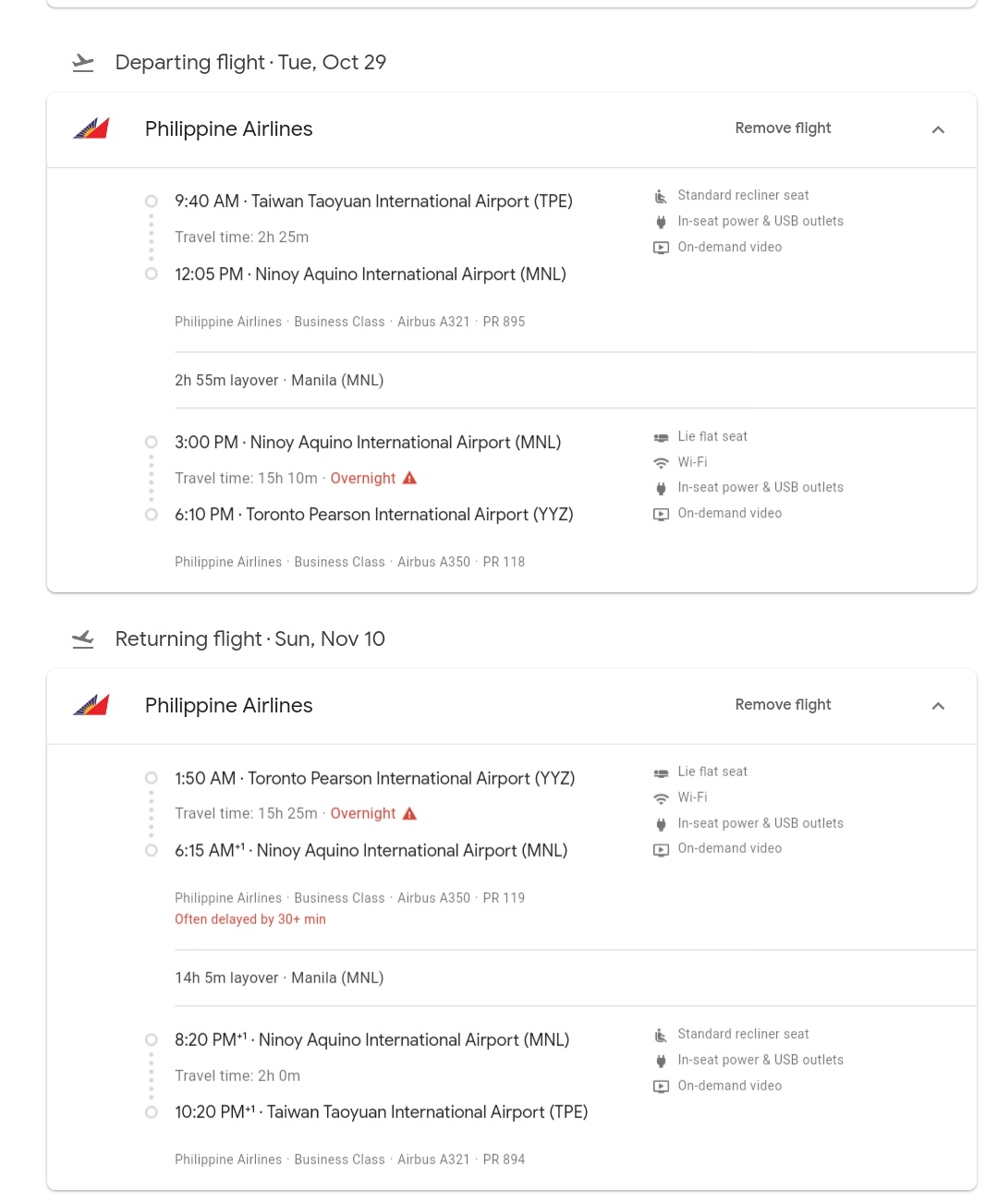A Philippine Airlines departing flight on Tuesday, October 29, showcased the airline’s Business Class service on an Airbus A321 (flight number PR895). The journey began at 4:00 AM from Taiwan Taoyuan International Airport (TPE), featuring standard reclined seats with in-seat power and USB outlets, as well as on-demand video entertainment.

The flight duration was 2 hours and 25 minutes, concluding at 12:05 PM at Ninoy Aquino International Airport in Manila. Subsequently, the travel continued with a layover, covering a total travel time of 15 hours and 10 minutes, and eventually arriving overnight at 4:00 PM in Toronto Pearson International Airport.

For the return journey, Philippine Airlines flight PR894 departed at 1:15 AM from Toronto Pearson International Airport and was scheduled to arrive back at Ninoy Aquino International Airport after a travel time of 15 hours and 25 minutes. This flight segment, often delayed by over 30 minutes, includes a 14-hour and 5-minute flight with a layover in Manila and a subsequent travel time of 2 hours to reach Taiwan Taoyuan International Airport by 10:20 PM.

The airline's Business Class on the Airbus A321 featured comfortable standard reclined seats equipped with in-seat power and USB outlets, alongside on-demand video services, ensuring a pleasant and connected flight experience.